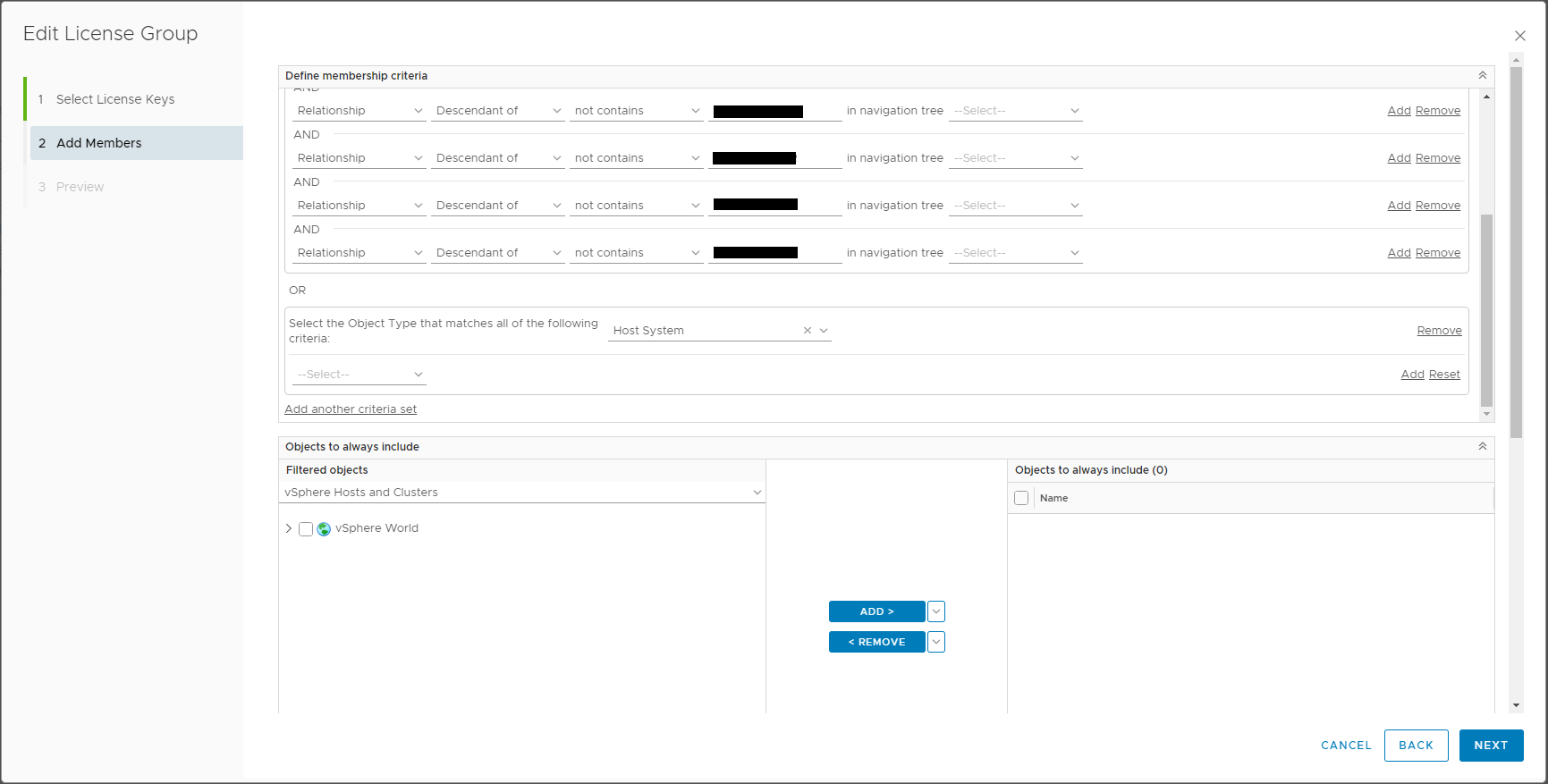**Caption:**

The screenshot depicts a WordPress content upload interface tailored for managing a license group. On the left pane, there's a title at the top left corner that reads "Edit License Group". Below the title, three rows are visible:

1. **Select License Keys**
2. **Add Members** (highlighted)
3. **Preview**

Adjacent to this pane is a vertical green line.

The right pane is dedicated to the "Add Members" section. It features two charts:

**First Chart: Define Membership Criteria** - This chart includes three repeating sections. Each section starts with a bubble labeled "Select the object type that matches all of the following," followed by criteria such as "Host Systems," "Relationships," and "Descendants of contains." Part of the criteria text has been redacted. Each section has an empty dropdown bar underneath the criteria.

**Second Chart: Objects to Always Include** - This chart has two panes:
- **Filtered Objects**: Features a checkbox labeled "vSphere World" accompanied by a globe icon.
- **Add/Remove Buttons**: Blue buttons for adding and removing objects.

To the right of this section is another area titled "Objects to Always Include" with a checkbox next to "Name."

At the bottom left corner of the screenshot, there are two buttons: a back button and a blue next button, alongside a cancel text option.